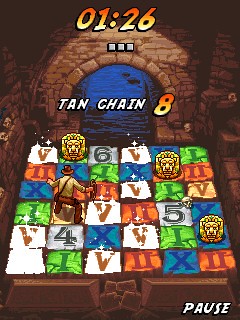This screen capture from a video game features a detailed and pixelated scene with an Indiana Jones theme. The lower half of the image displays a game board comprising 36 squares arranged in a grid, with five columns and six rows. Each square is variously colored and marked with Roman numerals, letters, or distinctive designs, such as gold lion heads. Standing in the second column of the third row from the bottom is a character resembling Indiana Jones, identifiable by his brown brimmed hat, tan long-sleeved shirt, brown pants, and a brown bag slung across his shoulder, with his back turned towards the viewer.

In the upper half of the image, there is a stone arch that appears tunnel-like, made of brown stone. Above this central area, the time "01:26" is prominently displayed in orange-yellow letters. Directly below the time, the overlay text "TAN CHAIN" is seen in white capital letters, accompanied by an adjacent "8" in reddish-yellow text. The image is set against a dark background, enhancing the visibility of the game's elements. In the lower-right corner, the overlay word "PAUSE" is written in white capital letters, indicating that the game is paused.